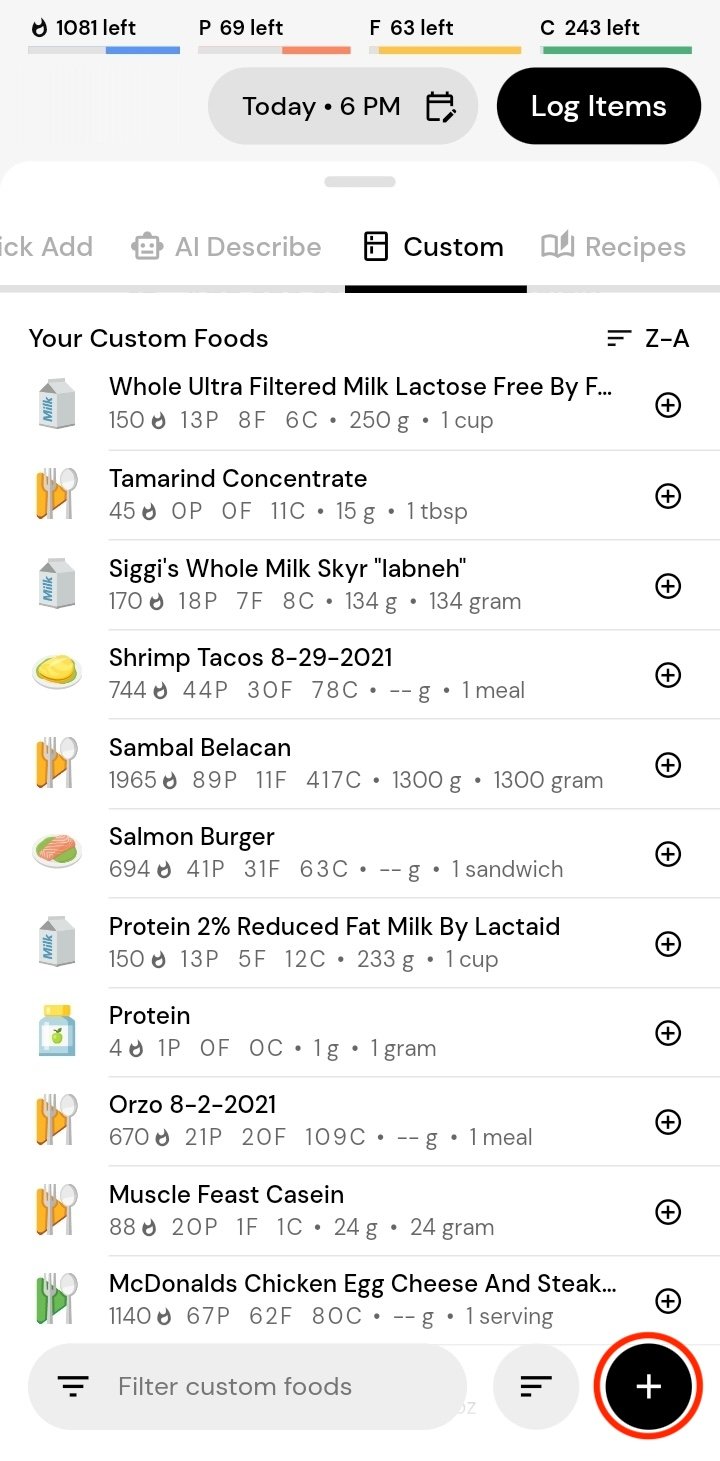This is an image of a computer page with distinct columns and various data entries. At the top, there are four columns displayed in black font. The first column reads "1081 left," the second column shows "P 69 left," the third says "F 63 left," and the fourth indicates "C 243 left." Each of these columns is underlined with colorful lines - blue, orange, yellow, and green, respectively.

Beneath these columns, there is a central box that states "today 6pm." To the right of this box, there's a black button featuring white text that reads "log items."

Below this section, several titles appear. The leftmost title is partially cut off, followed by "AI described," "custom," and "recipes."

Further down, there is a series of listings, each accompanied by an image. The listings are as follows:
1. Whole Ultra-Filtered Milk
2. Tamarind Concentrate
3. Siggy's Whole Milk
4. Shrimp Tacos
5. Sam Ball (spelled B-E-L-L-A-C-A-N)
6. Salmon Burgers
7. Protein 2% Reduced Fat Milk
8. Protein
9. Orzo 8-2-2021
10. Muscle Feast K-C-N-C-A-S-E-I-N
11. McDonald's Chicken, Egg, Cheese, and Steak

Each item on the list features a corresponding picture, adding a visual reference to the descriptive text.